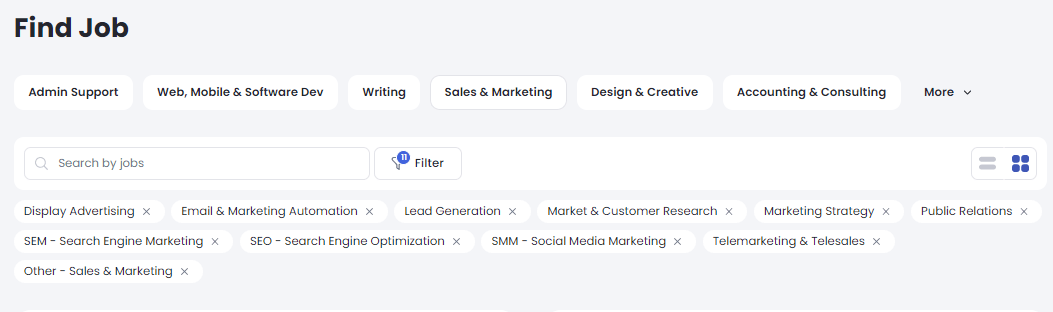In this horizontal, thin rectangular web interface, occupying less than half of a typical webpage, the top-left corner features the black text "Find Job." Directly beneath it spans a row of white buttons with black text, categorizing job types as follows: Admin Support, Web, Mobile, and Software Development, Writing, Sales and Marketing, Design and Creative, Accounting and Consulting, and More.

Below this button row, starting from the left, is a search bar labeled "Search by Jobs," accompanied by a filter button. 

Further down, there are three rows of tags, each denoting various job categories, with the final row comprising a single tag. From the top left, these tags include: Display Advertising, Email and Marketing Automation, Lead Generation, Marketing Customer Research, Marketing Strategy, Public Relations, SEM (Search Engine Marketing), SEO (Search Engine Optimization), SMM (Social Media Marketing), Telemarketing and Telesales, and Other Sales and Marketing.

Aligned with the search bar on its right side, there are two small square icons. One icon contains two grey lines, while the other features four blue squares, likely representing different view or filter options.